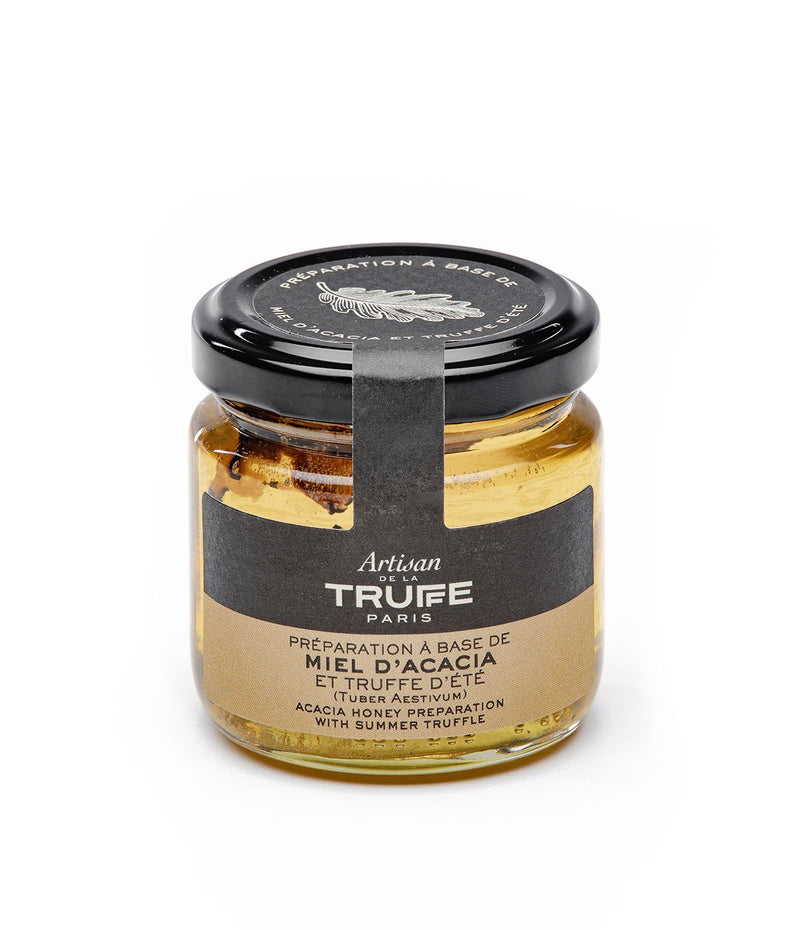This high-resolution product photograph features a clear jar of acacia honey with summer truffle, ideal for a catalog or advertisement. The jar has a black lid adorned with a drawing of a leaf in the center. A label extends from the black lid down the length of the jar, acting as a safety seal. The top half of the label is black with white text, reading "Artisan de la Truffe, Paris," while the bottom half is a cream or light brown color, inscribed with “Préparation à base de Miel d’Acacia et Truffe, TRUFFE d'Été (Tuber Aestivum).” The English translation at the very bottom states, "Acacia Honey Preparation with Summer Truffle." The jar contains light yellow honey with darker brown flecks, likely pieces of truffle, adding an artisanal touch to this luxury product. The entire image is set against a completely white background, ensuring full focus on the elegant and detailed jar.